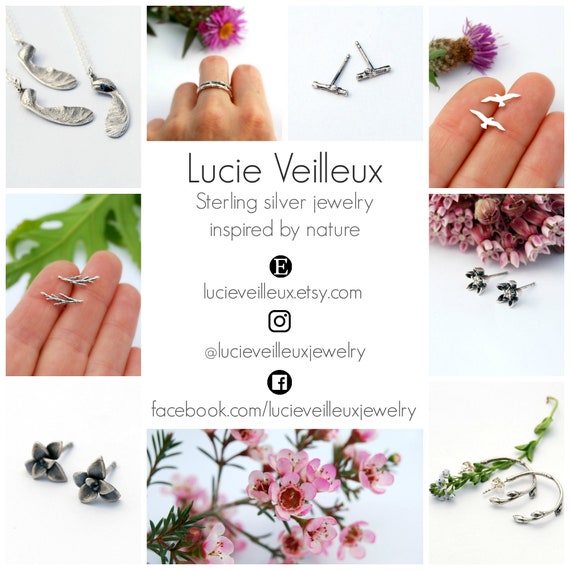The image is a detailed advertisement for Lucy Veloz's sterling silver jewelry, inspired by nature, featuring a mix of various natural elements and color schemes. At the center of the image is a white square with the text in black and gray that reads "Lucy Veloz Sterling Silver Jewelry Inspired by Nature." Surrounding this central text are multiple smaller square images against a clean white background.

On the top right, a white hand holds two little silver bird pendants alongside a flower. Below this are several silver pieces, including a silver ring set against pink and yellow flowers with green leaves. To the left, twig-shaped earrings can be seen in a white hand with a green leaf backdrop. The far-right square presents silver floral earrings with diamonds and pink flowers. Each piece of jewelry, whether earrings, rings, or necklaces, is carefully juxtaposed with flowers or held by hands, emphasizing an organic and nature-inspired aesthetic.

The colors featured throughout the advertisement range from subtle greens, blacks, pinks, reds, purples, whites, grays, to tan and beige. Additional contact details are provided below the central text, including a URL (lucyvelicks.etsy.com), and Instagram handle (@lucyvelicksjewelry), and a Facebook page (facebook.com/lucyvelicksjewelry). Each of these symbols and text are displayed in black and gray, maintaining the elegant and cohesive design of the advertisement.